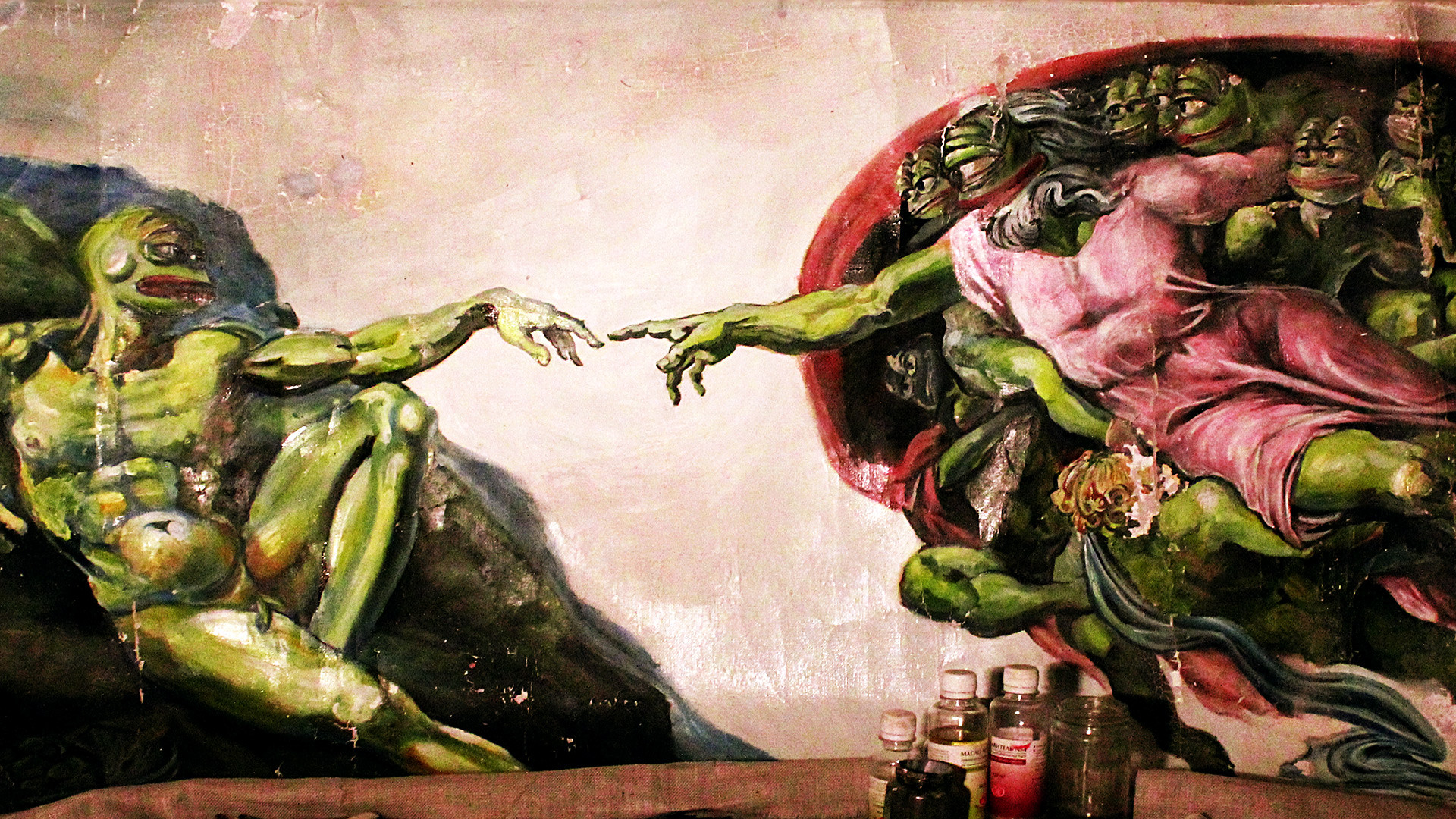In this tan-backed image, rendered in the style of a famous Renaissance painting, there are two central figures evocative of Michelangelo's "Creation of Adam." On the right, a seated, muscular green creature donning a rose-colored tunic sits on a green material embedded within an oval red outline. This figure's right arm is extended towards the figure on the left, with its index finger pointing. The right figure's head and face are partially covered. Surrounding this figure is a group of similarly green, frog-like beings who all gaze towards the left. The left figure, also a green creature, has frog-like features including bright red lips and saggy eyes. This figure reclines on a rock, mirroring the finger-reaching gesture towards the right. This alien-like form has one bent leg outlined distinctly, contributing to its buff, humanoid appearance. In the foreground, a brown wooden table holds five bottles of liquid, featuring labels in yellow and red-pink, with additional clear cups. The background behind the figures showcases a light brown shade blended with white, particularly in the central area, adding depth to the scene.